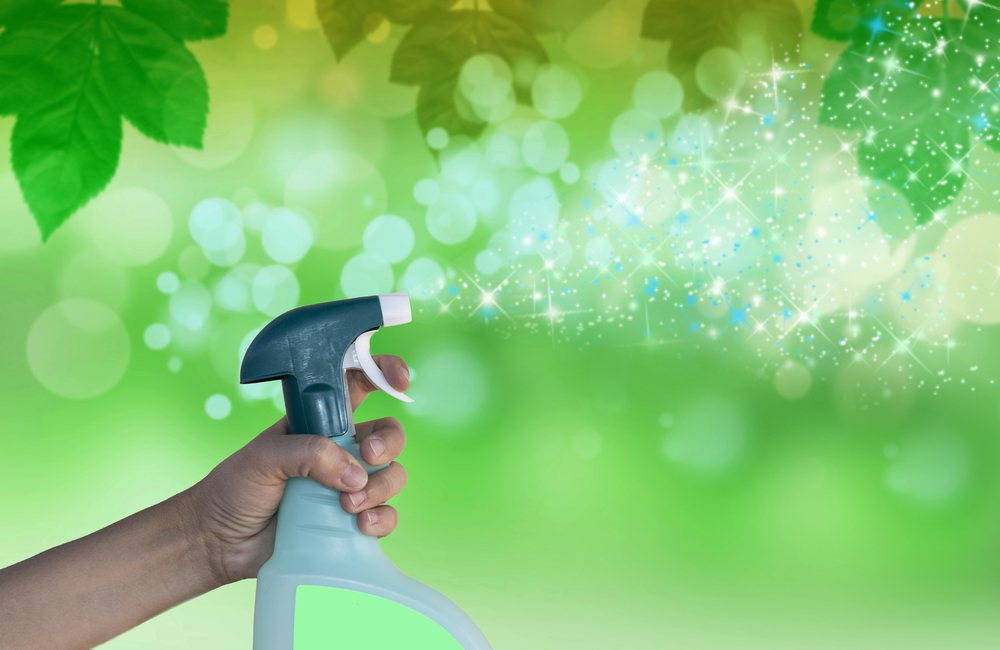This image features a cleaning product against a vibrant, cartoon-like background. The backdrop is a gradient of green shades with bokeh effects, characterized by large white and blue dots, and adorned with bright green leaves at the top corners, transitioning to darker green in the center. In the lower left-hand corner, a tan-skinned hand holds a spray cleaner, with fingers wrapped around its nozzle. The spray bottle has a blue or green head, a white nozzle tip, and a white trigger, while the body of the bottle is gray with an indistinct light green label. Animated twinkling bits, resembling glowing white and blue stars, emanate from the nozzle, enhancing the lively and whimsical feel of the image.